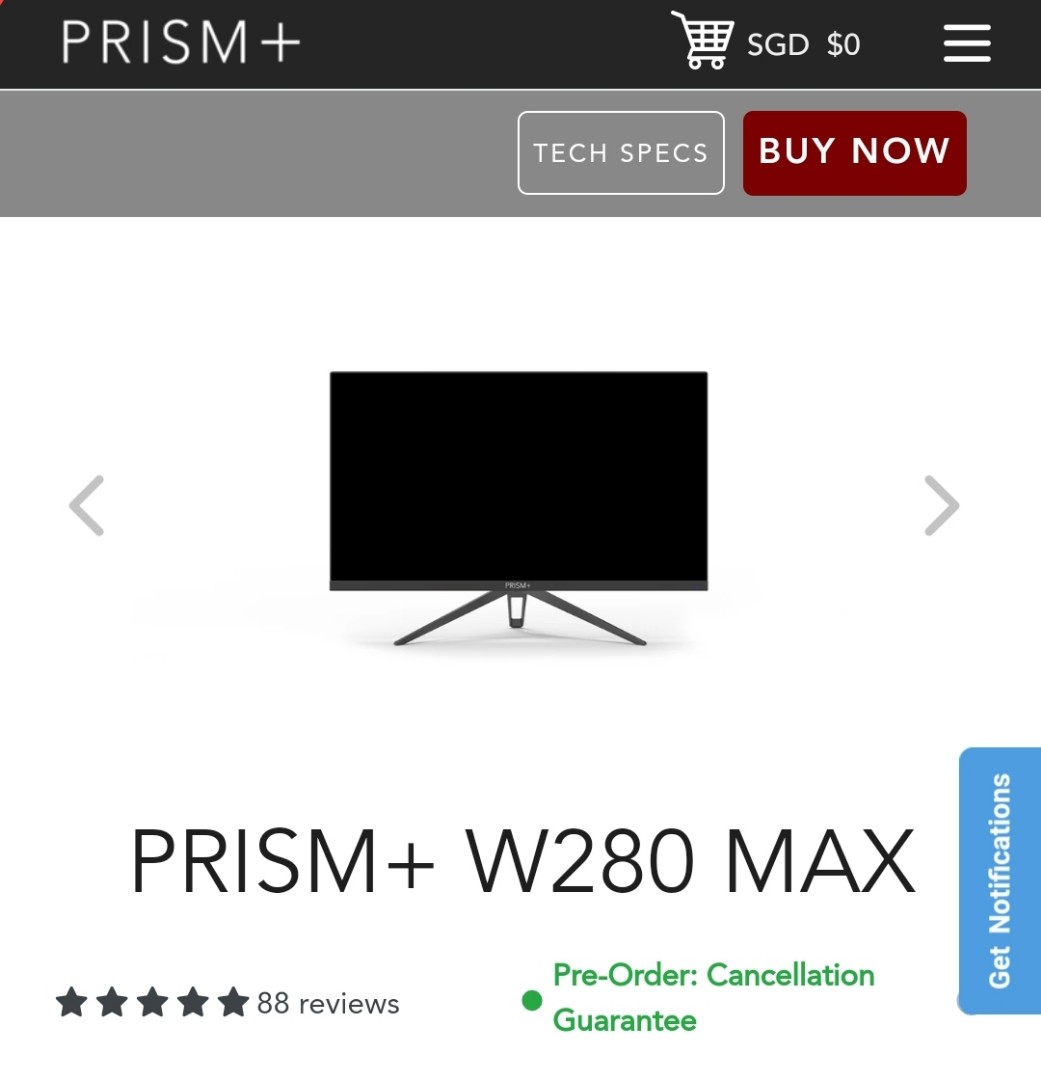Screenshot of a Shopping Cart Page on Prism Plus Website

The screenshot showcases the shopping cart section of the Prism Plus website. At the top, there's a prominent black banner featuring the "Prism Plus" logo in white on the left side. Adjacent to the logo, on the right side of the banner, there's a white shopping cart icon followed by an "SGD 0" label in white text. Next to this, there are three horizontal lines stacked vertically, indicating a menu or additional options.

Below this, a horizontal gray banner spans the page. On the far right of this banner, there are two buttons: a white-outlined gray button labeled "Tech Specs" in white text, and a maroon-colored button with "Buy Now" written in white.

The central portion of the screenshot displays an image of a black monitor mounted on a tripod stand. Flanking the monitor image, there are gray left and right arrows, allowing users to navigate through a gallery of images. Directly beneath the monitor image, the product title "Prism Plus W280 Max" is prominently displayed in black text. Below the product title, five solid black stars signify the product's rating, with an annotation indicating "88 reviews" to its right.

Additionally, to the right of the reviews, there's a green bullet point followed by the text "Pre-Order Cancellation Guarantee" in green, signifying a customer benefit. On the bottom right of the page, there is a vertical blue rectangular button with the text "Get Notifications" in white, suggesting that users can sign up for alerts or updates.